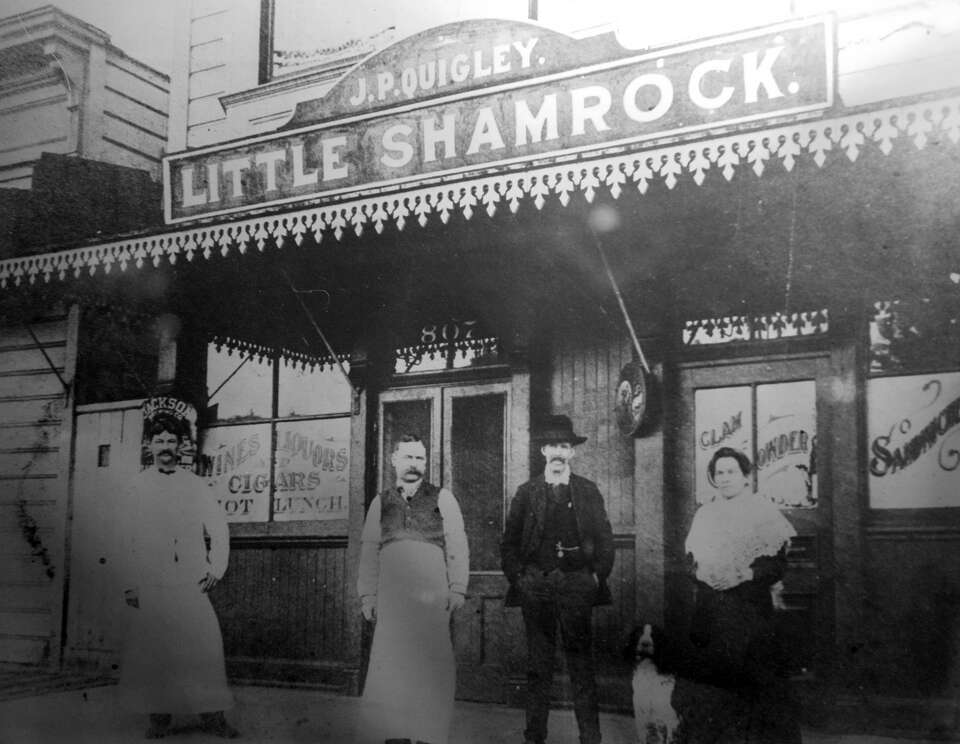This black and white photograph, likely taken in the 1800s, depicts an outdoor scene in front of J.P. Quigley's Little Shamrock at 807, a retail space that features signs advertising wines, liquors, cigars, and hot lunch, including clam chowder. The square image, which appears to be captured using natural light, shows four people and a dog. Under a hand-painted sign, three men and one woman pose in front of the establishment. Two men are dressed in long white aprons, suggesting they might be workers, while the third man, possibly the shop owner, wears a black suit and hat. The woman is attired in a black dress with a white top. Enhancing the vintage atmosphere, a dark and white dog lounges in the scene. The building, reminiscent of an old saloon, exudes a nostalgic charm with its wooden doors and classic signage.